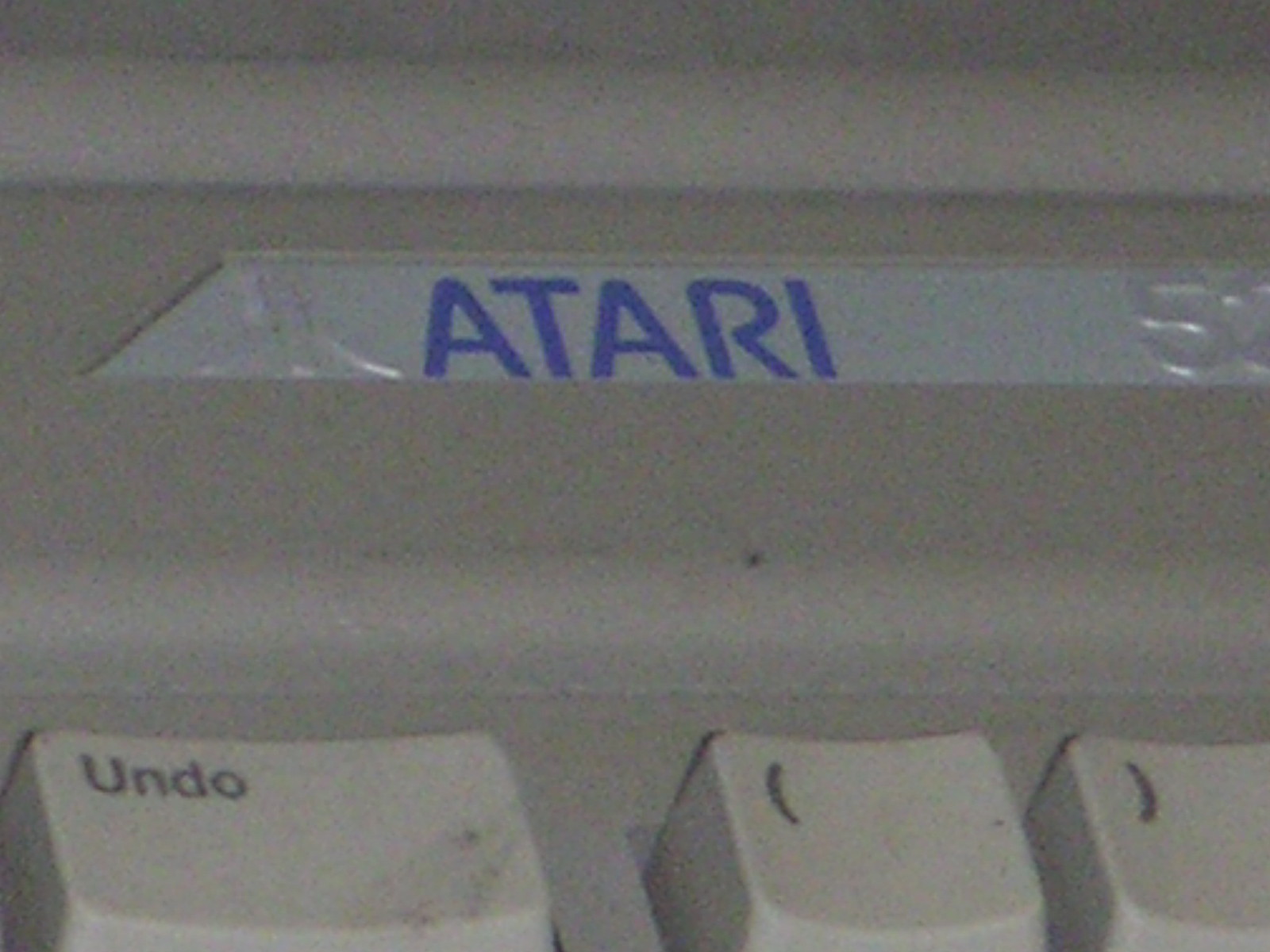A detailed caption for the image described:

"This close-up, color photograph showcases a vintage Atari computer system, prominently featuring a section of its keyboard and a part of its main console. The rectangular image, a bit wider than a standard desktop view, highlights the classic beige color scheme typical of old computer hardware. At the bottom of the frame, three keyboard keys are visible, with the leftmost key labeled 'UNDO' being slightly wider. To the right, there are two adjacent keys marked with left and right parenthesis symbols.

Moving upwards, a raised strip of the console is visible, still in beige, which includes a small fold or indentation at the top. Centrally located within this section, the name 'Atari' is emblazoned in blue on a metallic silver background, indicating a different material from the rest of the console. On the left side of this silver strip, the recognizable Atari logo is subtly embossed. Towards the far right end of this banner, a partial number '5' is discernible, with the rest of the text trailing off and becoming unclear."